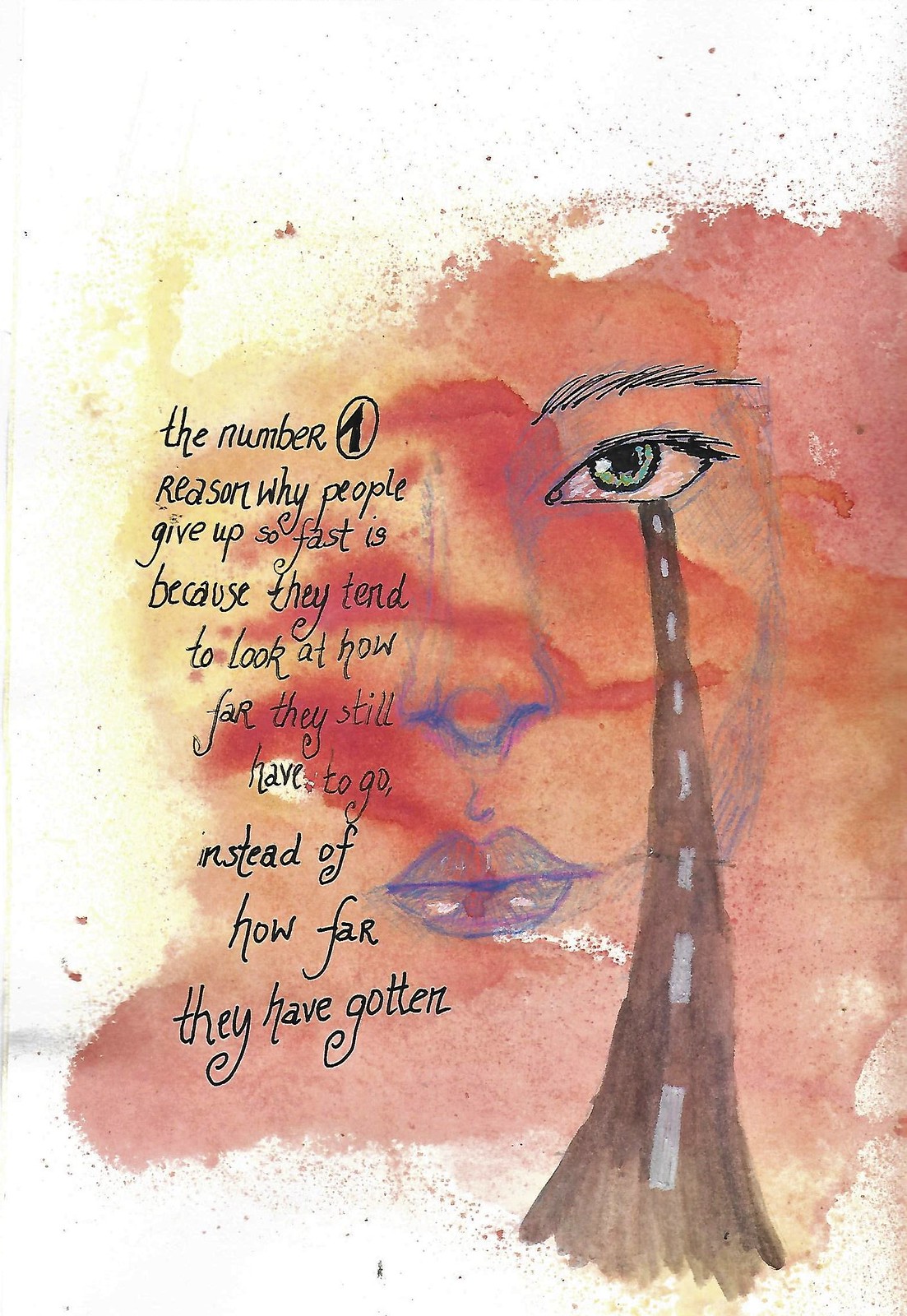The image is an inspirational poster featuring a watercolor depiction of a woman's face against the backdrop of a white canvas speckled with the paint used to create the portrait. The woman, painted in hues of browns, pinks, oranges, and yellows, has outlines of her face, nose, and lips sketched with a purply-blue pencil. Her expressive green eye, accentuated by a dark eyebrow, gazes out at the viewer. From her eye, much like a trail of tears, flows a brown-painted road with a white dotted line running down its center, leading towards the bottom of the image. Black handwritten-style text, though clearly added digitally, is positioned on the left side of the poster. It reads: "The number one reason why people give up so fast is because they tend to look at how far they still have to go instead of how far they have gotten."